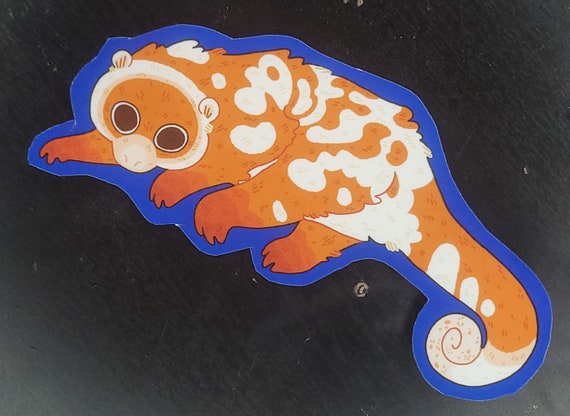The image depicts a colorful paper cutout of a creature, resembling a lemur or a monkey, placed on a black table. Captured from a top-down perspective, the cutout features a blue border, with an uneven, hand-cut edge. The creature itself is predominantly orange with irregular white spots and lines. Its face is highlighted by a white border, a white snout, and small white ears at the top of its head. Prominent brown eyes with white outlines give it a striking appearance. The creature has four legs and a distinctive long, curling tail that starts orange with white spots and ends with a completely white tip, curled towards the bottom right of the image. The head of the creature is positioned in the upper left corner, while the tail stretches towards the lower right corner. The cutout seems to have been crafted from paper or cardboard, underlining its homemade, arts-and-crafts feel.